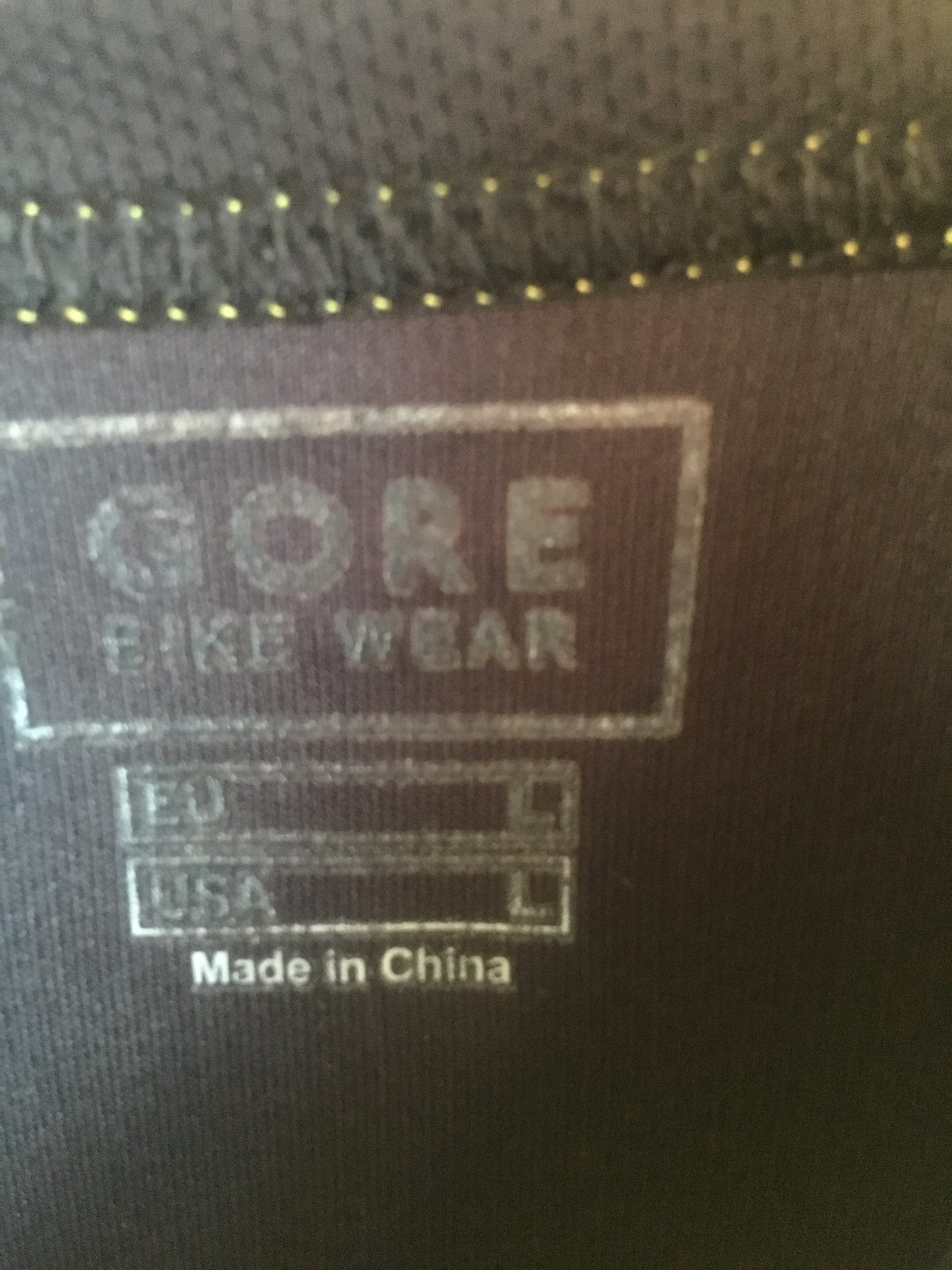The image depicts the interior labeling of a garment, likely a piece of bike wear, possibly a shirt or a coat. The label positioned at the collar area reads "Gore Bike Wear" in slightly faded, silverish-white lettering. Below this, size information is displayed as "EU L" and "USA L." A golden "Made in China" is also visible. The fabric of the garment appears to be a purplish-red, and the label is accentuated with distinct black stitching and a gold trim. The area around the label resembles a tag, but instead, it has white roping. Additionally, there's black knitting around the collar region, though the specific type of bike wear remains undetermined due to the close-up nature of the image.